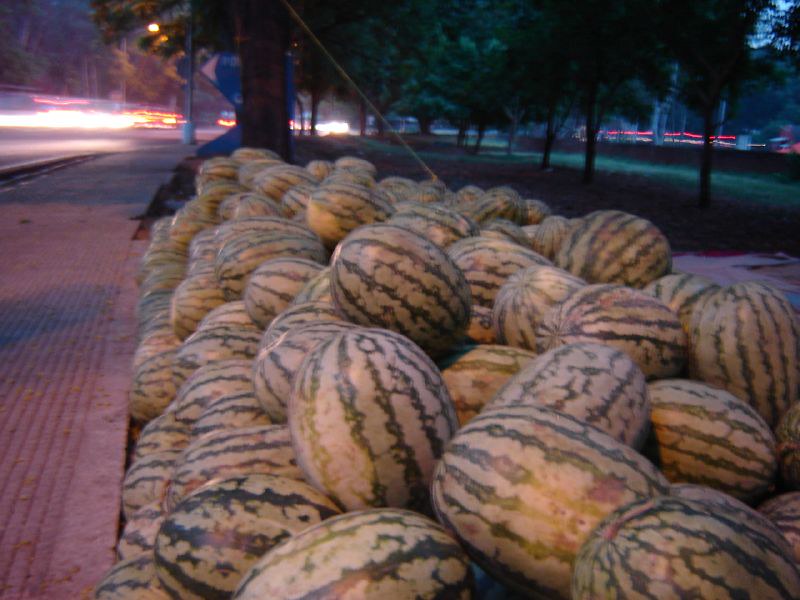In the foreground of this early evening outdoor color photograph, a substantial collection of freshly picked watermelons is prominently displayed. These ripe, oval-shaped melons—totaling around a hundred—are characterized by their distinctive green and tan stripes and are piled up in various positions along a red brick sidewalk, which stretches from the lower left corner up towards the center of the image. The red brick path continues to the left and beyond the frame, suggesting a long walkway. Adjacent to this path, a street is visible in the upper left corner, where blurred white streaks from car headlights indicate a time-lapse effect, capturing the motion of vehicles.

To the right and slightly in the background, a grass field dotted with about five to six tall, leafy trees can be seen, accentuating the summer season. Behind the field, a faint outline of a short building—a convenience store, perhaps—is visible, recognizable by its red neon stripe. The scene evokes a street market ambiance, with the meticulously stacked watermelons suggesting a roadside stand. The overall setting, with the street, sidewalk, and distant traffic lights, together with the abundance of melons, paints a vivid picture of a vibrant, bustling locale transitioning from day to night.